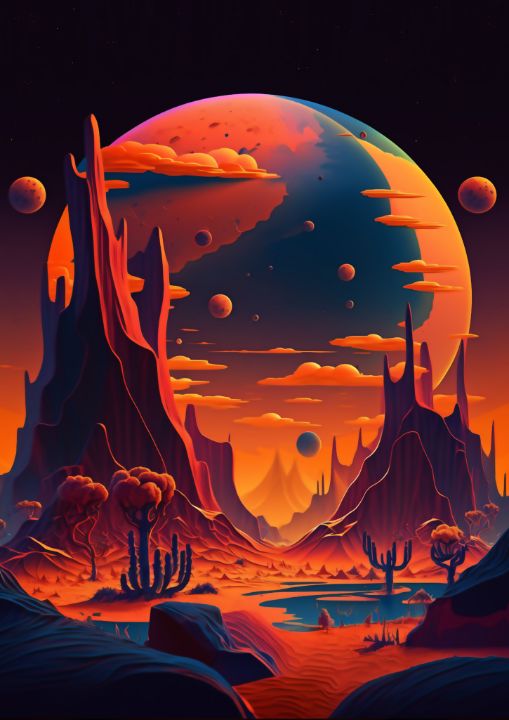This illustration portrays an enigmatic, otherworldly landscape teeming with vivid, contrasting hues. The vertically-oriented poster showcases a rugged, desert-like terrain dominated by dark blues, blacks, and vibrant oranges and reds. The ground is a tapestry of blue rocky zones, interspersed with bold red and orange sandy areas. Dotting the lower portion of the image are peculiar cactus-like plants with dark blue stalks crowned by red, bushy tops. A serene, bluish-green body of water nestles to the right, with an isolated cactus situated on a small island within. 

Towering rock formations, jagged and spiky, soar into the sky, cloaked in shadows that render them almost black, though some elements are distinctly red or dark blue. The sky above is a deep black canvas sprinkled with a plethora of planets—some orange, some blue—accentuated by a dominant large planet in the center, swirling with blue and orange hues and shrouds of orange clouds. The top of the poster captures a stark contrast with the dark void of space, highlighting the celestial bodies that dot the alien sky. The absence of text keeps the viewer's focus on the intricately detailed and animated depiction of this mythical planet, evoking the sense of an extraordinary, alien universe.